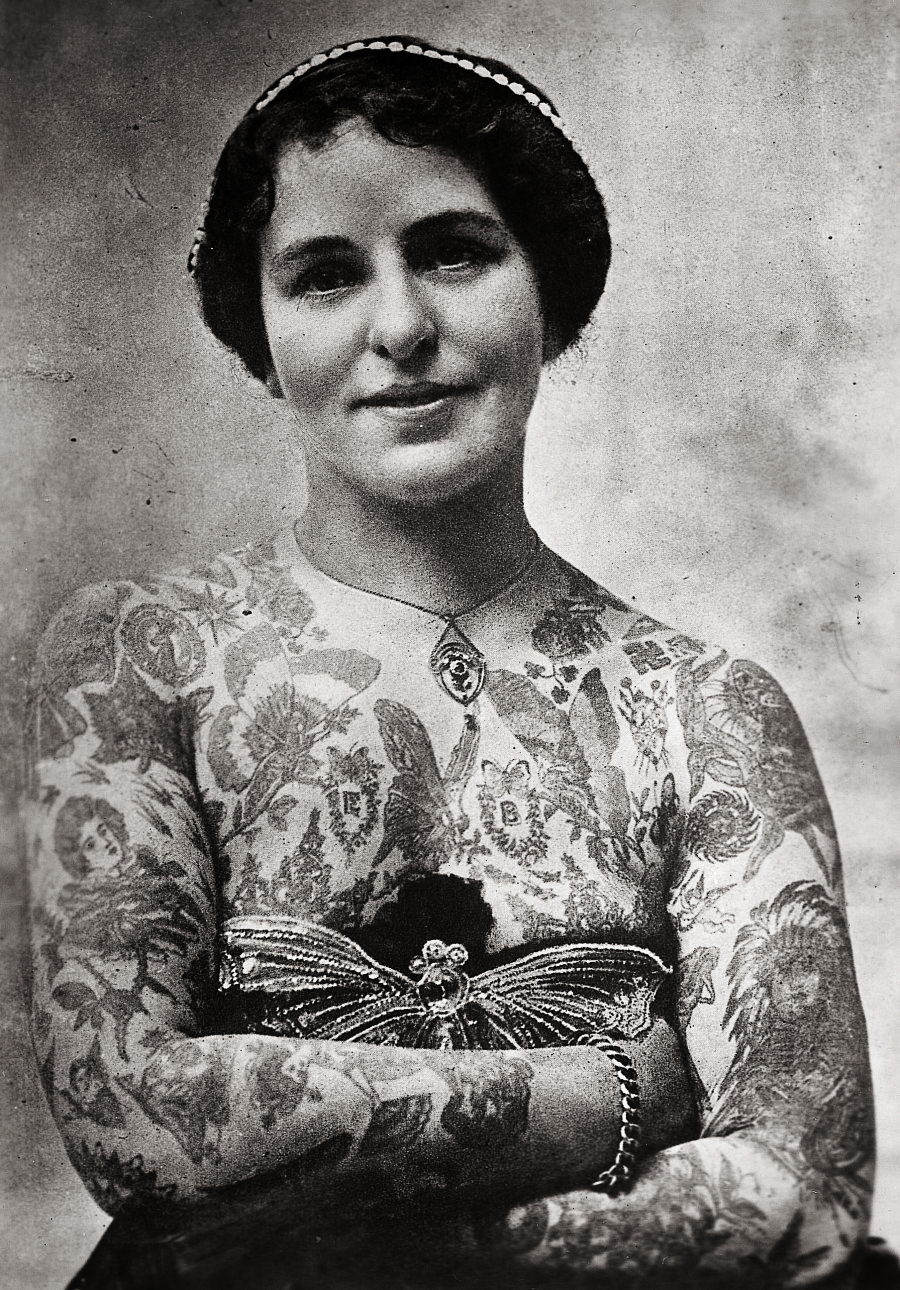In this vintage black and white photograph, a woman with light skin and a round face gazes directly at the camera, offering a slight, enigmatic smile. Her short black hair is adorned with a small hat or beret, and it appears to be held in place by a white headband. The photograph's background is a stark, grayish texture, emphasizing the central figure. She is dressed in a high-collared blouse, intricately patterned with motifs of butterflies and portraits. Her arms are crossed over her chest, with her right arm projecting slightly outward. Nestled between her arms, she clasps a large, reflective butterfly or moth-like brooch, which might also resemble a portion of her dress. Adding to her delicate ensemble, she wears a piece of jewelry on her right wrist, possibly a bracelet. The overall composition, marked by the photo's monochrome tones, underscores a sense of timeless elegance and mystery.